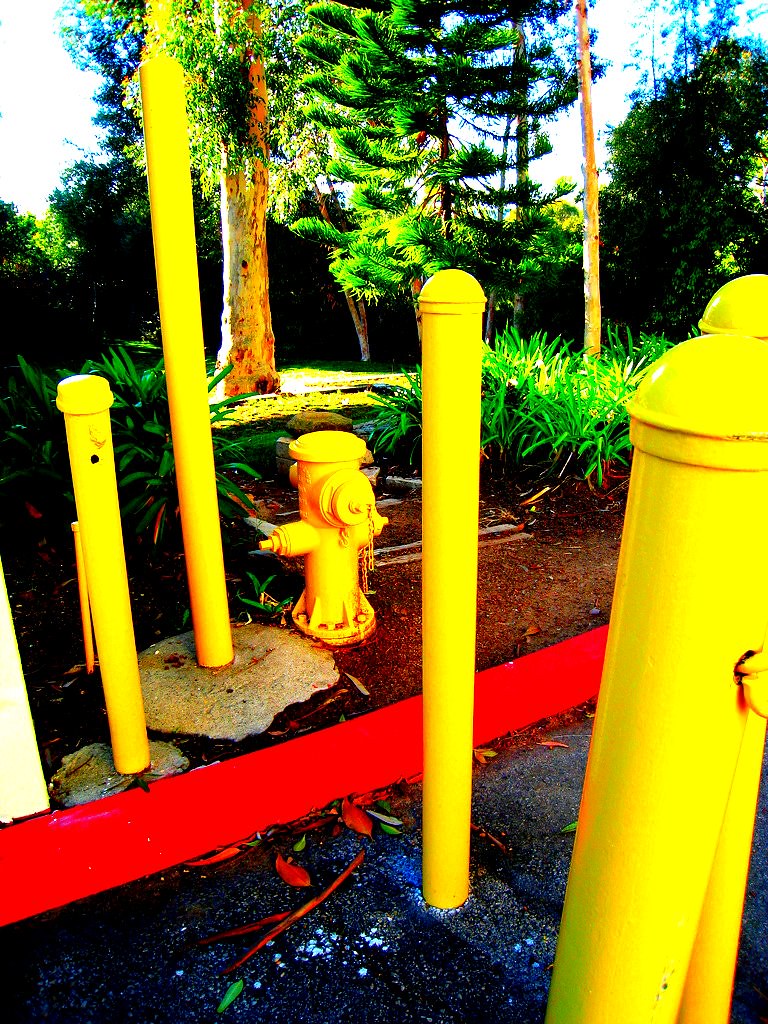The photograph depicts an outdoor scene characterized by extreme color saturation, creating an almost surreal vibrancy. Central to the image is a yellow fire hydrant surrounded by five similarly bright yellow metal poles of varying heights, each anchored into what appears to be a black concrete or tarmac surface. The fire hydrant and poles feature such intense yellow hues that they seem almost painful to look at. At the base of this setup, there's a strikingly vivid red kerb that contrasts sharply against the grey and blue tones of the surrounding ground surface.

In the background, lush greenery dominates, with a prominent conifer tree displaying a thick brown trunk and bushy foliage. The tree's leaves, as well as the other greenery in the scene, appear unnaturally vibrant due to the edited color balance, resulting in shades of green that are unusually bright. Smaller bushes and protruding branches further fill the scene, enhancing the image's dense, verdant atmosphere. The overall lighting suggests a sunny day, which accentuates the hyper-saturated colors and the high contrast created by the photograph's post-processing. In some parts of the image, the ground appears to have scattered branches, adding a touch of nature's randomness to the otherwise strikingly vibrant scene.